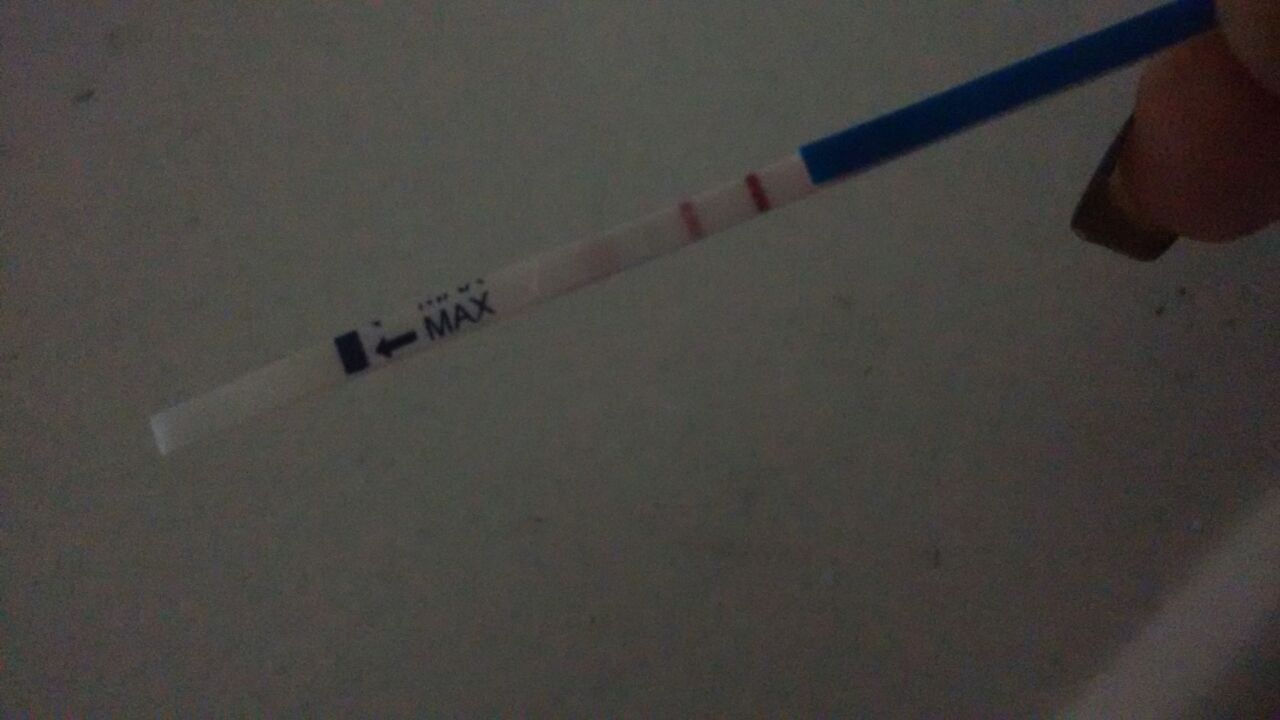The image depicts a medicine dropper being held by a person, similar to how one might hold a paintbrush. The person's middle finger is visible on the far right-hand side of the image. The dropper extends diagonally from the upper right corner down to the lower left, ending about a third of the way from the bottom and almost reaching the left edge of the frame. The handle of the dropper, which the person is gripping, is blue for approximately the first two-fifths of its length, followed by a section that appears to be made of either white or transparent plastic. Close to the blue portion, there are a couple of red lines. Further down, about two-thirds of the way along the dropper, the word "MAX" is printed in blue capital letters. To the left of the "MAX" label, there is an arrow pointing towards a rectangular marking.